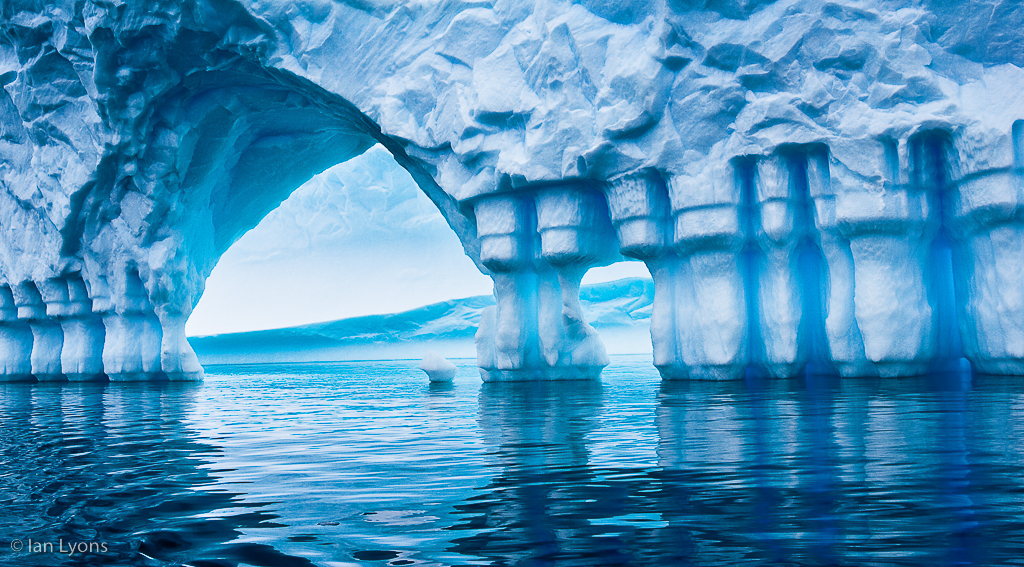The image depicts a stunning, computer-generated scene of a large chunk of ice arching over an icy-blue body of water. This arch-like glacier is supported by symmetrical, segmented pillars of ice and snow, which appear to be meticulously designed, giving them an unnatural, almost architectural quality. The crystal blue water below reflects light, enhancing the surreal beauty of the scene. In the distance, snow-capped mountains rise under a mostly white sky tinged with light blue at the top, suggesting daylight. A small piece of snow rests calmly on the water under the arch. In the lower left-hand corner, the name "Ian Lyons" is visible, likely identifying the creator or photographer of this visually striking image.